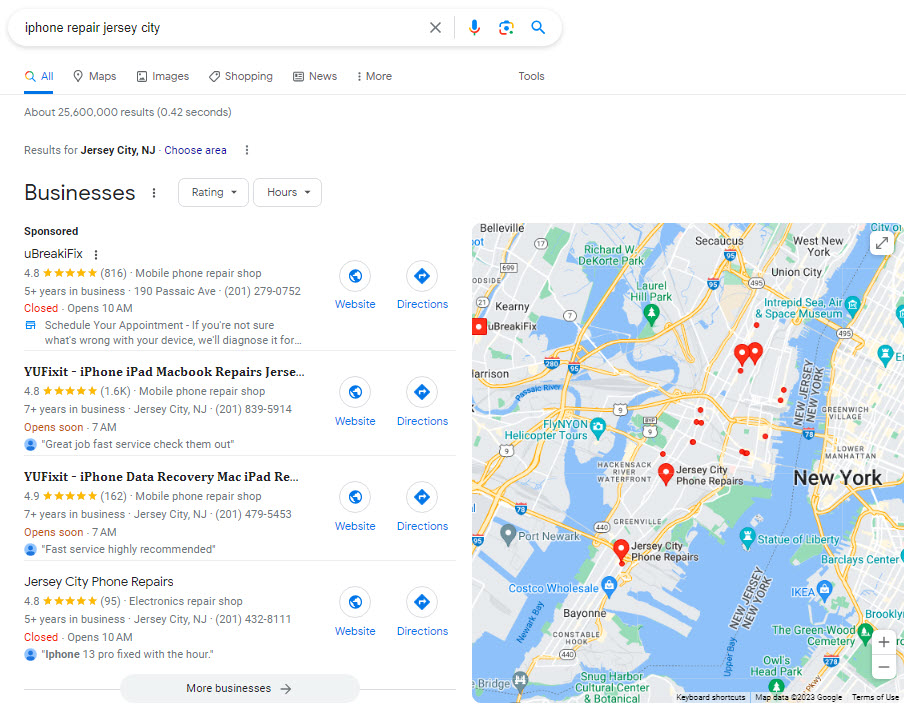The image depicts a Google search results page for "iPhone Repair Jersey City." In the top left-hand corner, there's a search bar displaying the entered query. Below the search bar is a list of several repair businesses, including 'You Break iFix,' 'Why You Fix It iPhone, iPad, MacBook Repairs,' and 'Jersey City Phone Repairs.' Each business listing features links to their respective websites and direction options. On the right side of the page, a map is visible, showing part of New York and New Jersey. The various repair business locations are marked with red balloon-like pins. The map clearly demarcates the areas labeled as New York and New Jersey. The background of the webpage is predominantly white, offering a clean and straightforward interface.